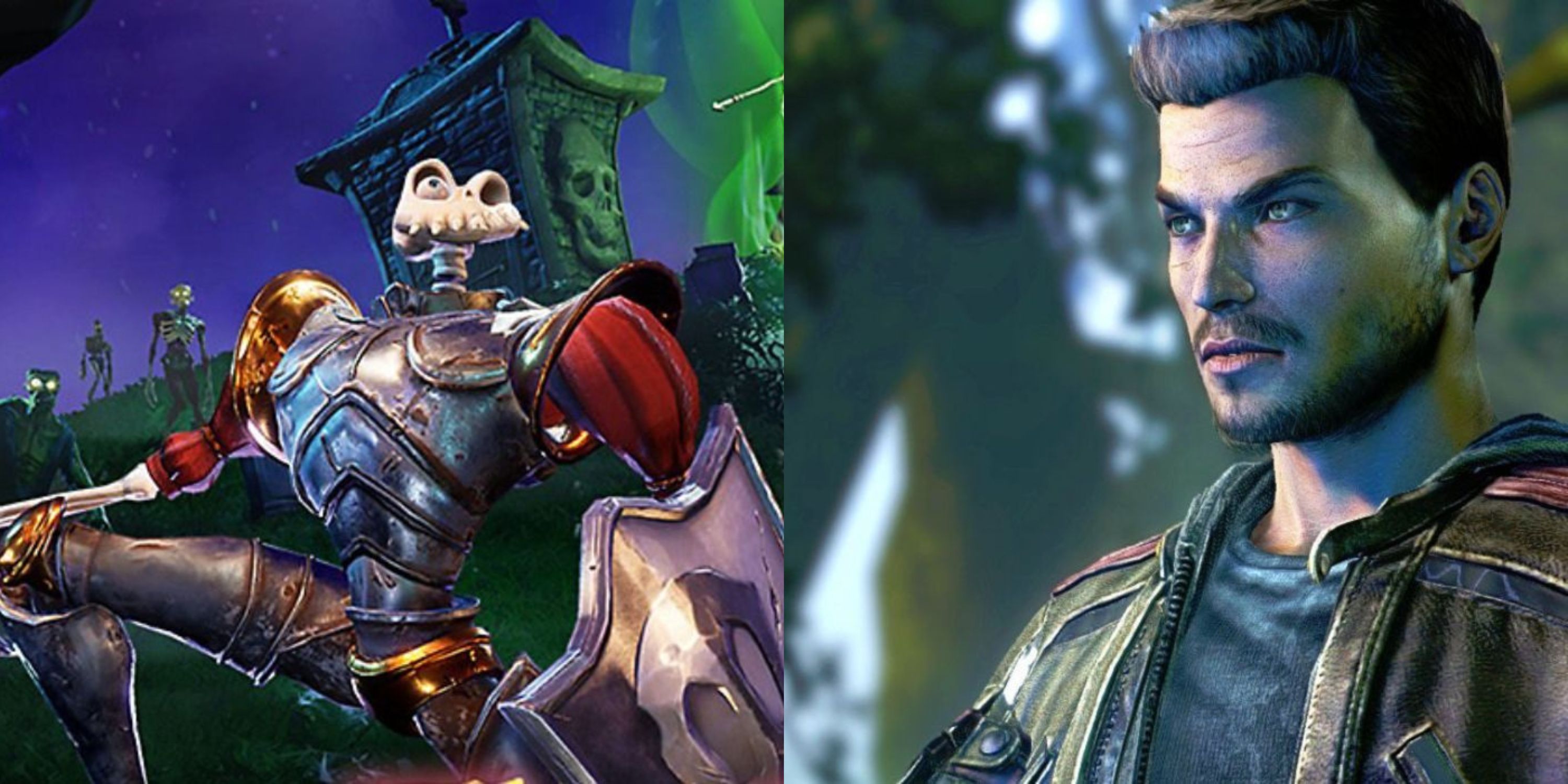This image is a digitally created, horizontally rectangular composition split down the middle into two vertically rectangular sections, each featuring distinct video game characters, and variegated with a rich palette of blue, green, red, black, gold, silver, and purple hues.

On the right side, the image showcases a detailed portrait of a young man. He sports a well-groomed appearance with a dark crew cut and a light beard. His intense gaze is directed towards the left, complimented by his attire—a blue t-shirt underneath a brown leather jacket. The colors and textures highlight the realistic quality of the character.

Contrastingly, the left side of the image is centered around a skeletal warrior adorned in battle armor, exuding a haunting presence. The skeleton is missing its lower jaw and one eye, presenting an intimidating visage. Clad in silver armor with red sleeves, it wields a silver shield. The background features a crypt set against a mysteriously dark and purple sky. Other zombie-like skeleton figures stand to its right and to the left on a grassy hill, enhancing the eerie, nightmarish atmosphere of the scene.

Together, these two images juxtapose the lifelike and the undead, creating a visually striking and detailed representation of diverse video game characters.